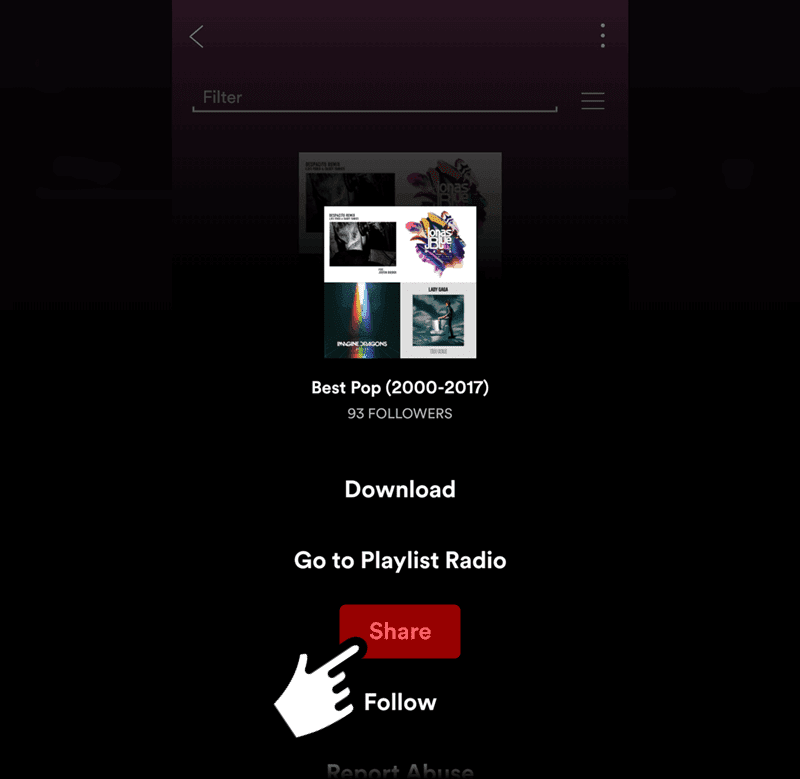The image showcases a social media profile related to music. Prominently displayed in the center is the title "Best Pop (2000-2017)" with an accompanying detail indicating "93 followers." Below this text, there are two options in white writing: a "Download" button and "Go to Playlist Radio." 

A red share button with pink lettering stands out, being clicked by a white hand outlined in black. Beneath this button, the word "Follow" appears in bold white letters. The background of the image is predominantly black, providing a stark contrast that highlights the text and buttons.

Above the title "Best Pop (2000-2017)," four small and blurry album covers are faintly visible, though they are not clear enough to discern specific details. At the very top of the image, the word "Filter" is displayed, followed by a thin horizontal line and three stacked lines that likely suggest a clickable menu for further options.

At the bottom, partially obscuring the text, the phrase "Report Abuse" is visible in white, hinting at the image's origin or the way it was cropped.